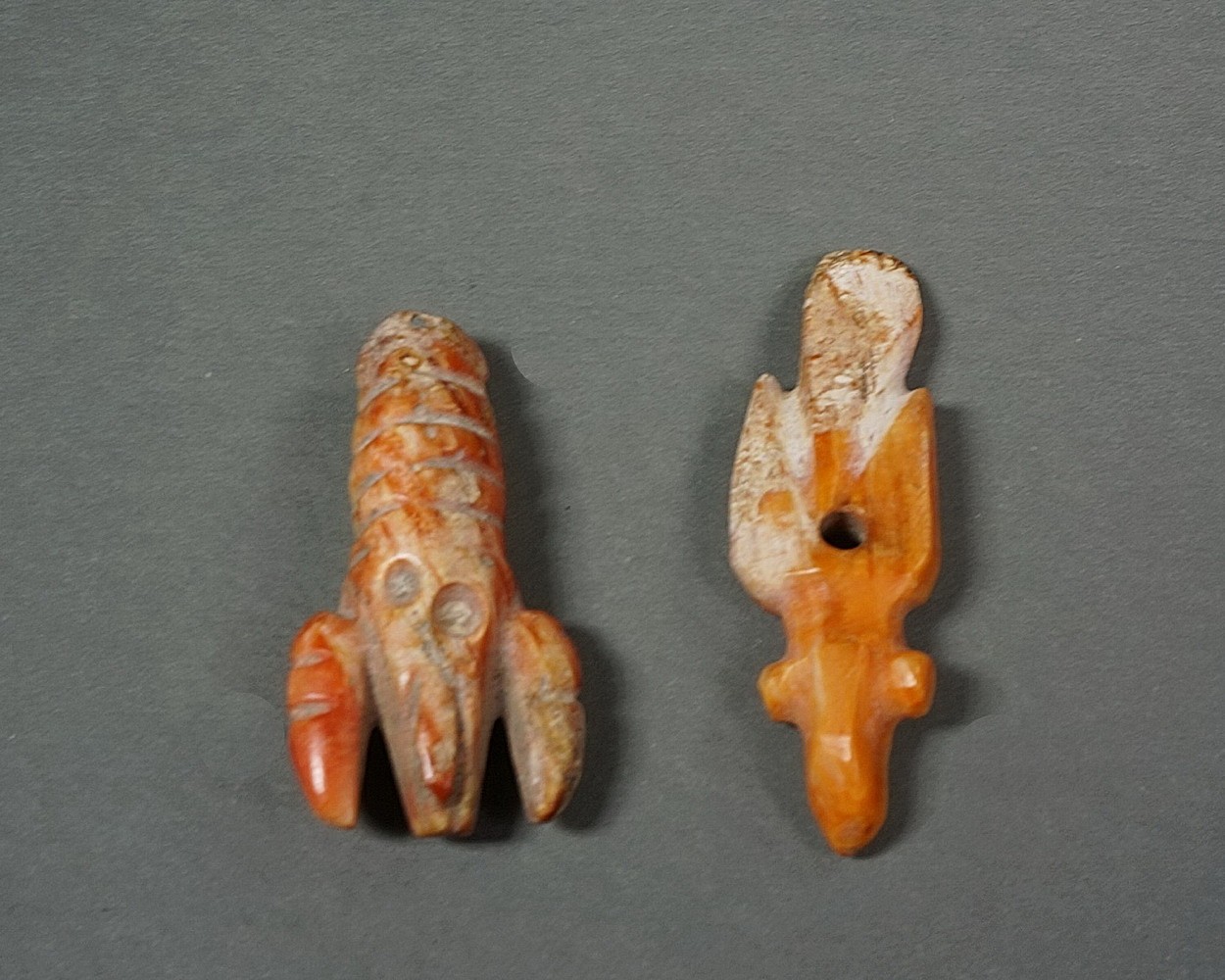This photograph features two vertically oriented, aged wood carvings placed on a dark gray background. Both carvings are slightly out of focus but display polished surfaces despite evident signs of wear and age, such as chips and faded areas. The carving on the left, with a reddish-orange hue, intricately resembles a lobster. It has distinct features including two indented eyes, a well-polished left claw, and several segmented sections trailing down its body. The right-hand carving is golden-tan and does not closely resemble any specific animal. It features a long, narrow head with a hole in the center of a rounded, paddle-like section beneath it, tapering into a cross shape. This piece also shows white streaks and signs of damage, emphasizing its antiquity.